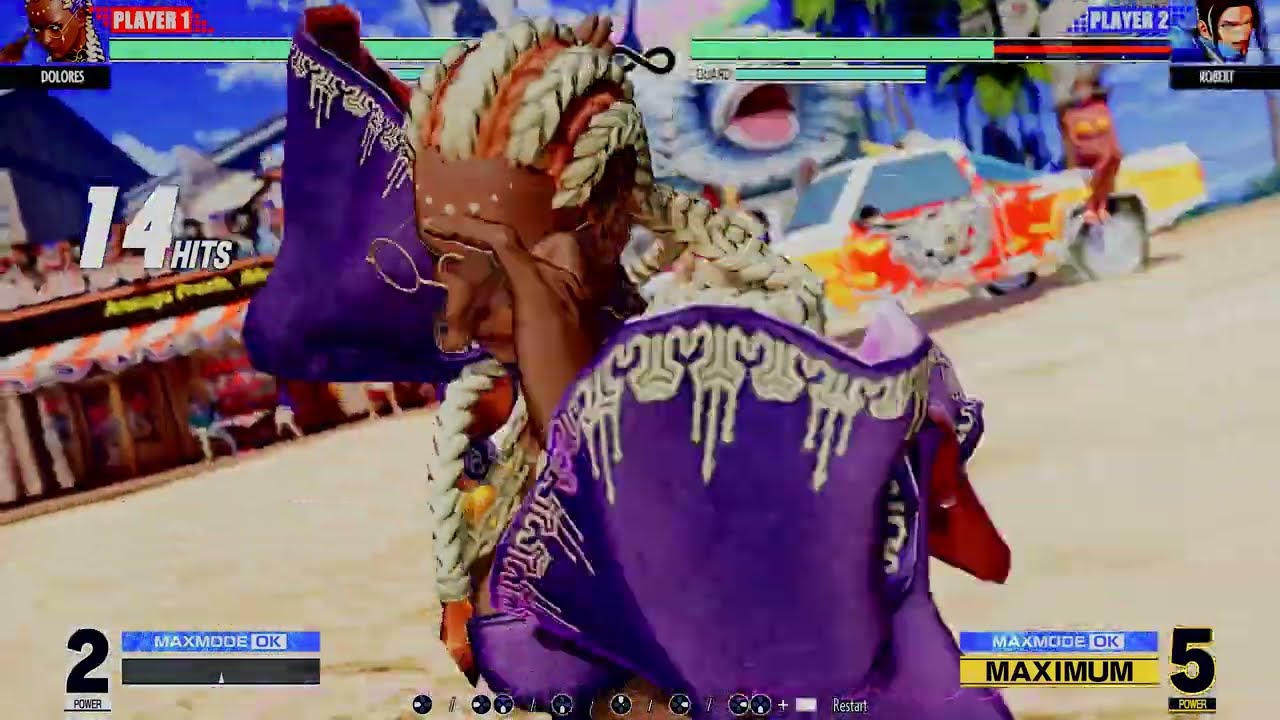In this video game image, the central character is a dark-skinned individual with mocha-colored skin, wearing thin, wiry gold-framed spectacles that they are adjusting. They have intricately braided hair threaded with gold and orange, and wear a vibrant purple outfit adorned with golden patterns, suggesting a prominent use of the color gold. The character's outfit includes a hood and appears to be somewhat baggy, with some white designs and an orange inner lining. The setting appears to be outdoors, featuring a bustling background with a red-and-white awning, a storefront with people walking around, and a yellow pickup truck with flame-like red designs and a white top. To the left of the character, an interface indicates "player one" and "player two," with green progress bars and various colored labels, including "max mode" and "power" indicators. Additionally, a "max mode okay maximum five" is displayed in the bottom right-hand corner, with the text "14 hits" positioned above the awning.